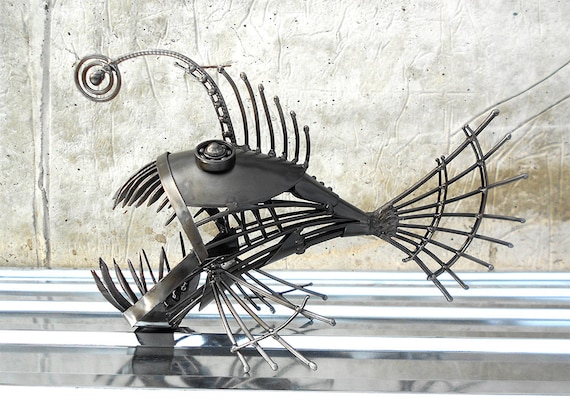This photograph showcases an intricate modern art installation of an anglerfish, crafted entirely from various pieces of metallic material, accentuating a steampunk vibe. The sculpture is highly detailed, featuring a wireframe body that skillfully simulates the fish's skeletal structure. The head of the anglerfish faces left, with nuts and bolts ingeniously integrated to form its eyes. Its gaping mouth reveals sharp, metallic teeth, adding to the ominous appearance. Above the mouth, a distinct metallic appendage mimics the anglerfish's bioluminescent lure.

The fish's midsection is an open wireframe, providing a clear view of its intricate internal metal framework. The tail fans out elegantly to the right, also formed from entwined metal wires. This sculpture sits upon a surface that appears to be a reflective metal or glass table, supported by metallic bars, and surrounded by a pristine, white backdrop. The setting's clean, industrial aesthetic is punctuated by what seems to be a cement wall in the background, suggesting an ambiguous indoor or outdoor location. The overall monochromatic color scheme, featuring dark and light gray tones, highlights the raw, mechanized beauty of the artwork.